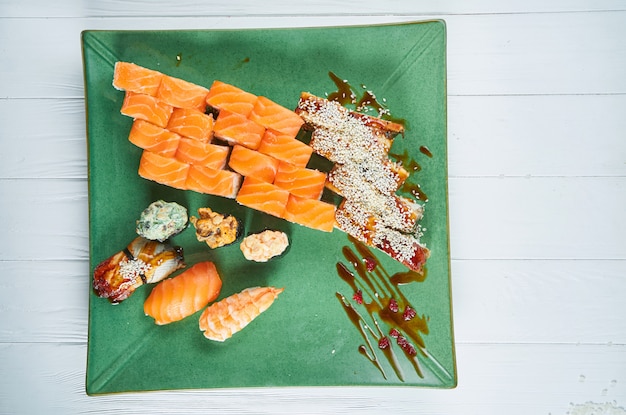This is a highly detailed photograph depicting a square teal glass plate meticulously arranged on a white, wooden table. The plate, slanted slightly to the left, holds an assortment of sushi pieces, varying in types and colors. There are around 16 to 18 pieces, including several with salmon on top, some colored coral, light blue, tan, and white. A few pieces appear to have a light white powder, possibly salt, sprinkled on top. Among them, there are pieces resembling shrimp and others that are more decorative in appearance. Drizzled across the plate is a swirled pattern of sauce, adding an artistic touch to the composition. The overall presentation is both visually appealing and slightly ambiguous, resembling a realistic painting.